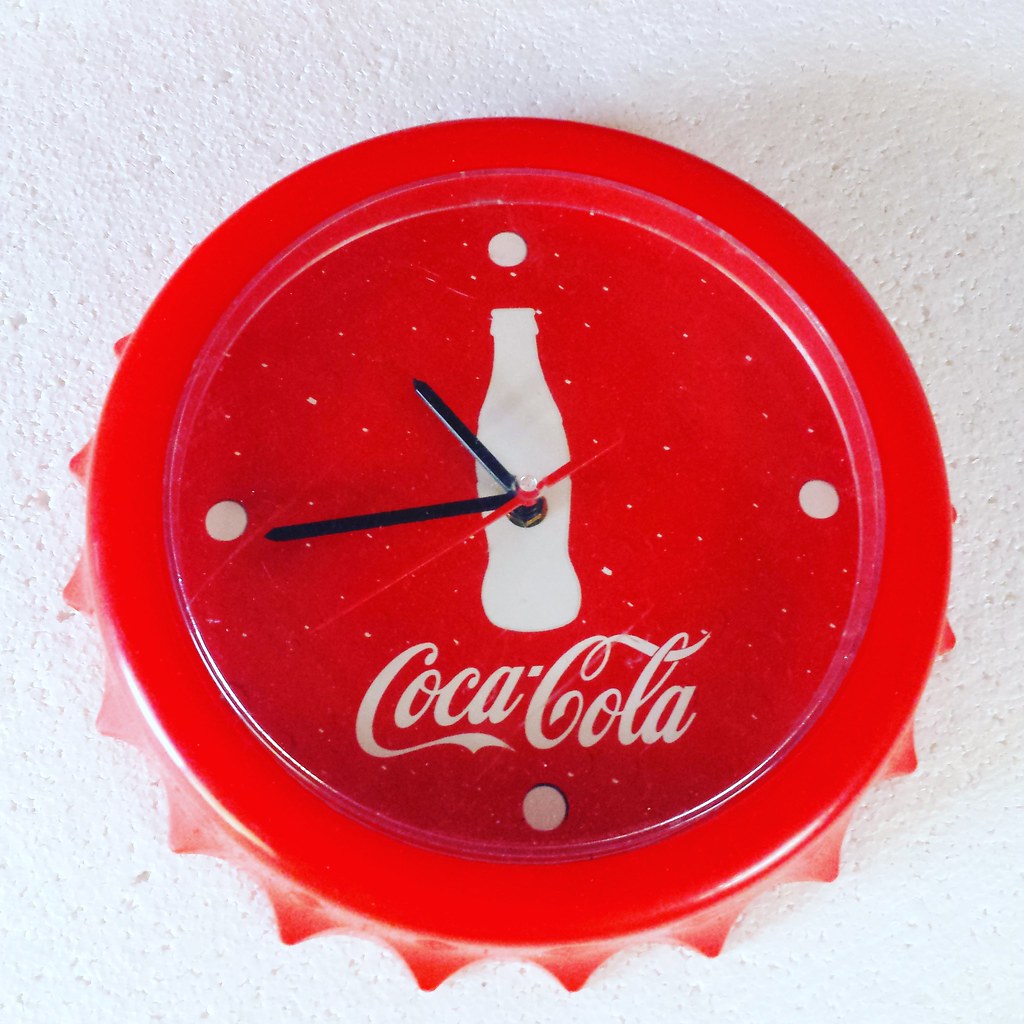The photograph features a distinctive Coca-Cola-themed clock mounted on a textured white wall. The circular clock is designed to resemble a bottle cap, with sharp, ridged edges around its red border. The clock face is also red and lacks numerical markers, instead displaying four prominent white dots at the 12 o'clock, 3 o'clock, 6 o'clock, and 9 o'clock positions. The time-telling hands include two black arms for the hours and minutes, as well as a thin red hand for the seconds.

At the center of the clock face, a white silhouette of a Coca-Cola bottle stands out, with the clock hands emerging from its base. Beneath this bottle silhouette, the iconic Coca-Cola logo is prominently displayed in its classic cursive font. The surface of the clock face appears to have some white specks or chip marks, adding to its vintage charm. The clock’s unique design and attention to detail make it an eye-catching piece that adds a nostalgic touch to any setting.